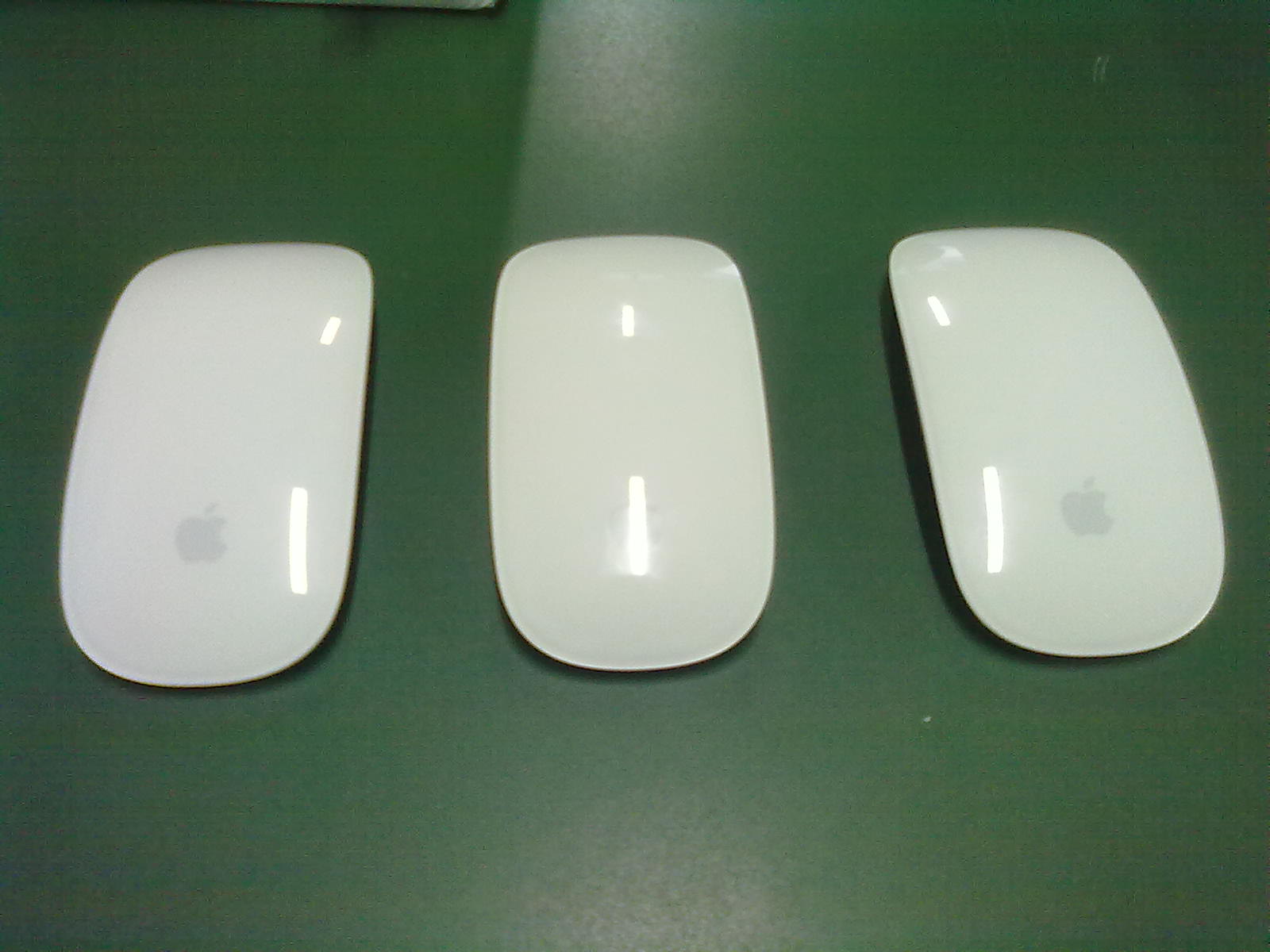This close-up photograph captures three thin, curved Apple mice aligned side-by-side on a dark green, shiny surface, possibly vinyl or another polished material. Each mouse is glossy white and features the iconic Apple logo—a small silhouette of an apple with a floating stem and a bite taken out of the right side—positioned towards the front bottom. The central mouse's logo is partially obscured by a bright reflection from overhead fluorescent lighting, while the right side of the table adds a subtle glow. The reflective nature of the mice reveals lines of light across their surfaces, especially noticeable with the central and right mice. The overall image is illuminated from above, with lighting reflections enhancing the white gloss of the Apple mice and casting subtle highlights on the dark green tabletop.